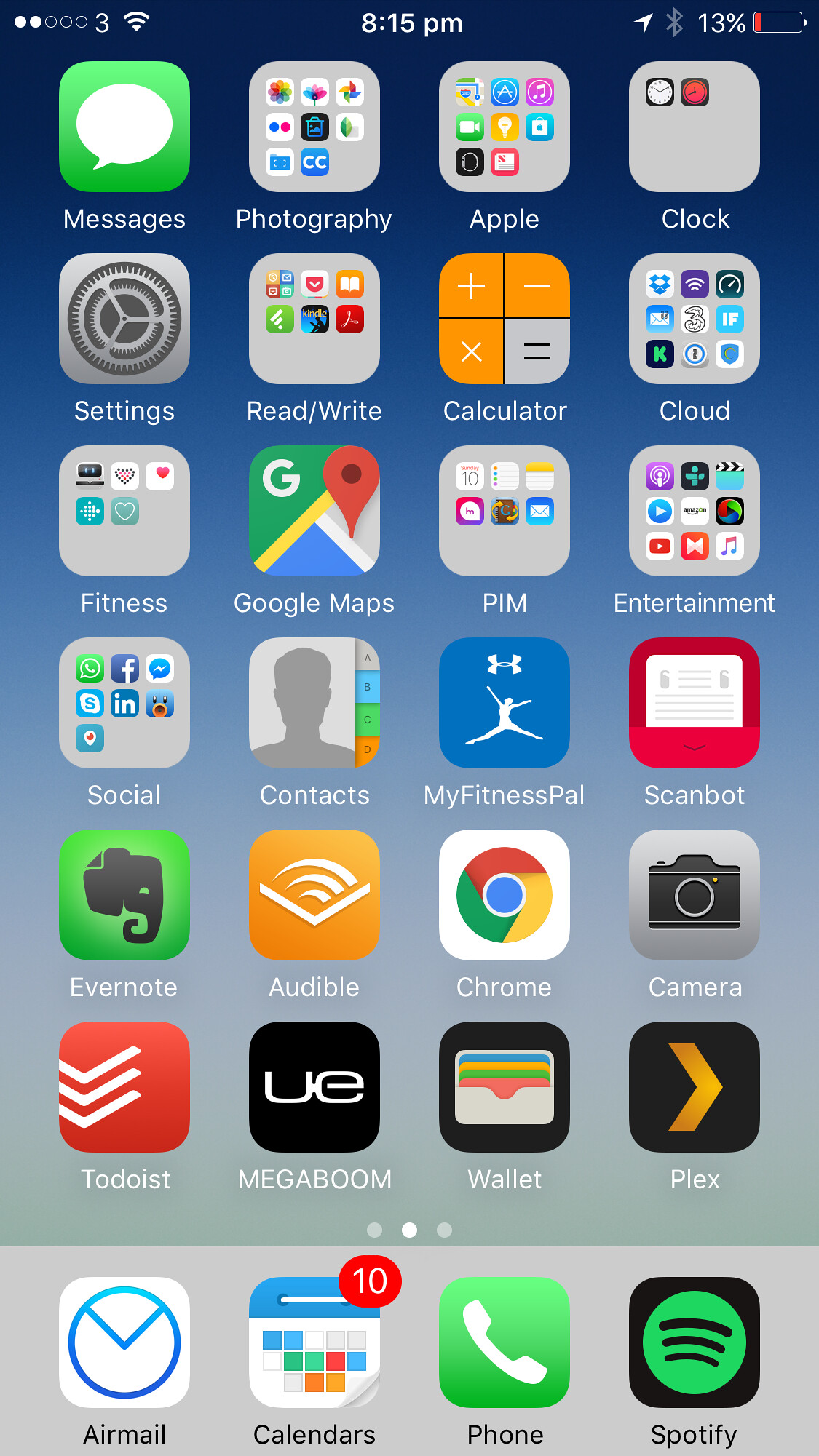Screenshot of an iPhone home screen displaying various apps organized into categories and rows. The time is shown at the top of the screen, reading 8:15 PM, with a battery level at 13%. 

The screen is organized as follows:

- **Top Status Bar:** Displays the time, battery level, and an iPhone message icon.
- **Apps Overview:**
  - **Bottom Row (Docked Apps):** Air Mail, Calendar, Phone, and Spotify.
  - **Top Row:** Photography collection, Apple apps collection, and Clock.
  - **Second Row:** Settings, Read and Write category, Calculator, and Cloud category.
  - **Third Row:** Fitness category, Google Maps category, Personal Information Management (PIM) category, and Entertainment category.
  - **Fourth Row:** Social category, Contacts, MyFitnessPal, and Scanbot.
  - **Fifth Row:** Evernote, Audible, Chrome, and Camera.
  - **Sixth Row:** To-Do List, Megaboom, Wallet, and Plex.

The apps are meticulously organized to showcase diverse functionalities from productivity and navigation to fitness and entertainment.